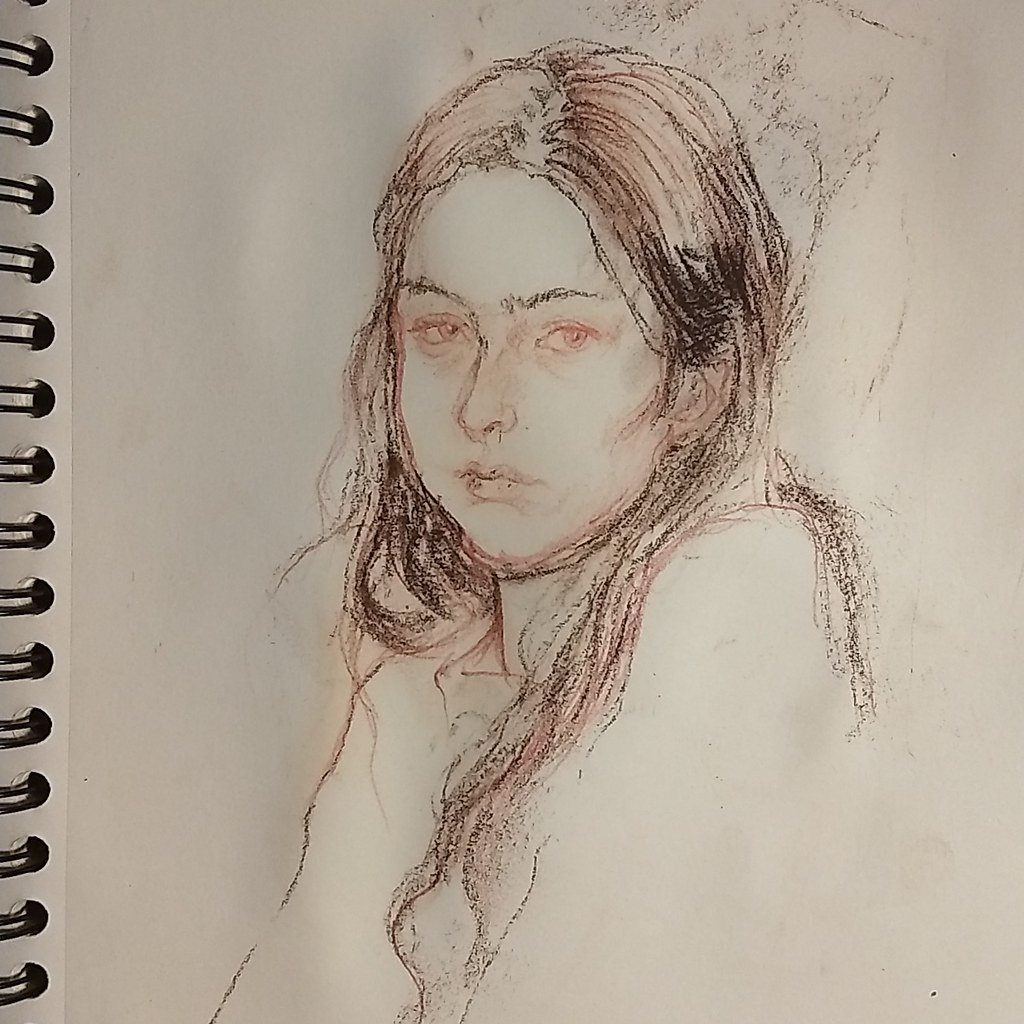This image showcases a meticulously detailed pencil sketch on white paper, captured within a spiral sketchbook, evidenced by the visible metal rings along the left edge. The artwork features a strikingly sad woman with long, light brown hair that drapes over her shoulder, partially covering her chest. Her hair, parted and intricately rendered, reveals individual pencil markings highlighting its delicate texture. The woman's face is depicted head-on, accentuating her somber expression. Her eyes, tinted with a light shade of red and meticulously outlined, convey a deep sense of sadness. She has thin black eyebrows and a closed mouth with faint brown speckles, adding to the melancholy aura. Her weak chin and frowning lips further emphasize her downhearted demeanor. She appears to be wearing a long-sleeved garment, possibly a turtleneck or jacket, as suggested by the outline of her shoulders and the subtle detailing at the neck's base. The careful shading and fine details in the sketch collectively capture the poignant essence of the subject.